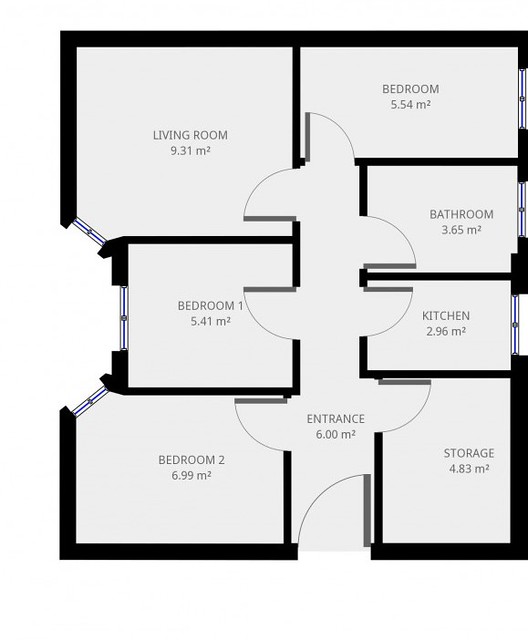This detailed blueprint illustrates the layout of a house or apartment, meticulously outlining each room's dimensions and arrangement within a rectangular structure. From the top moving left to right, the layout begins with a living room measuring 9.31 square meters. Adjacent to the living room is Bedroom 1, covering 5.41 square meters. Continuing along, there is a second bedroom, occupying 5.54 square meters, followed by a bathroom of 3.65 square meters. The kitchen, sized at 2.96 square meters, is also part of this efficient layout. Bedroom 2 is the largest sleeping area, featuring 6.99 square meters. The entrance or hallway spans 6 square meters, effectively connecting the spaces. Additionally, a dedicated storage area of 4.83 square meters ensures ample room for organization. Each room is marked with clear doorways, indicating the specific direction in which the doors swing open, depicted through a curved arc symbol. Overall, this schematic offers a comprehensive view of the living space's design and room-to-room flow.